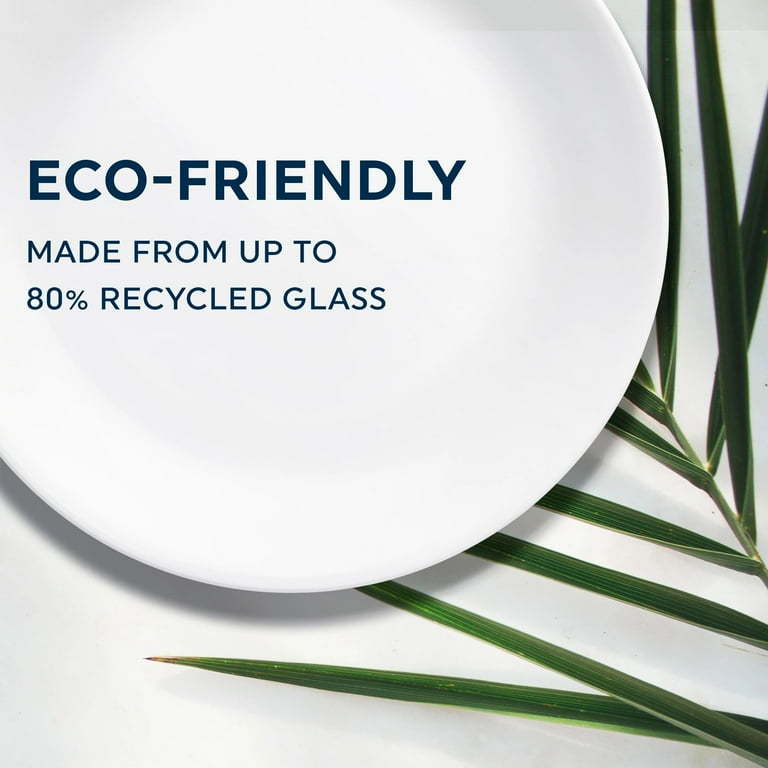The image features a white backdrop and showcases an arrangement emphasizing eco-friendliness and simplicity. Dominating the upper left corner is a pristine, white dinner plate, made from up to 80% recycled glass, as stated in blue text on the plate. The text reads: "Eco-Friendly, made from up to 80% recycled glass." The plate appears to be floating above a white surface. Adding a touch of nature, a long, green fern leaf with pointed tips extends from the bottom right corner, curving gracefully around to partly obscure the plate. This sparse but vivid leaf enhances the natural, eco-conscious aesthetic of the scene. The overall composition, set within a rectangular frame, merges clean white and lush green elements to underscore themes of environmental sustainability and minimalistic design.